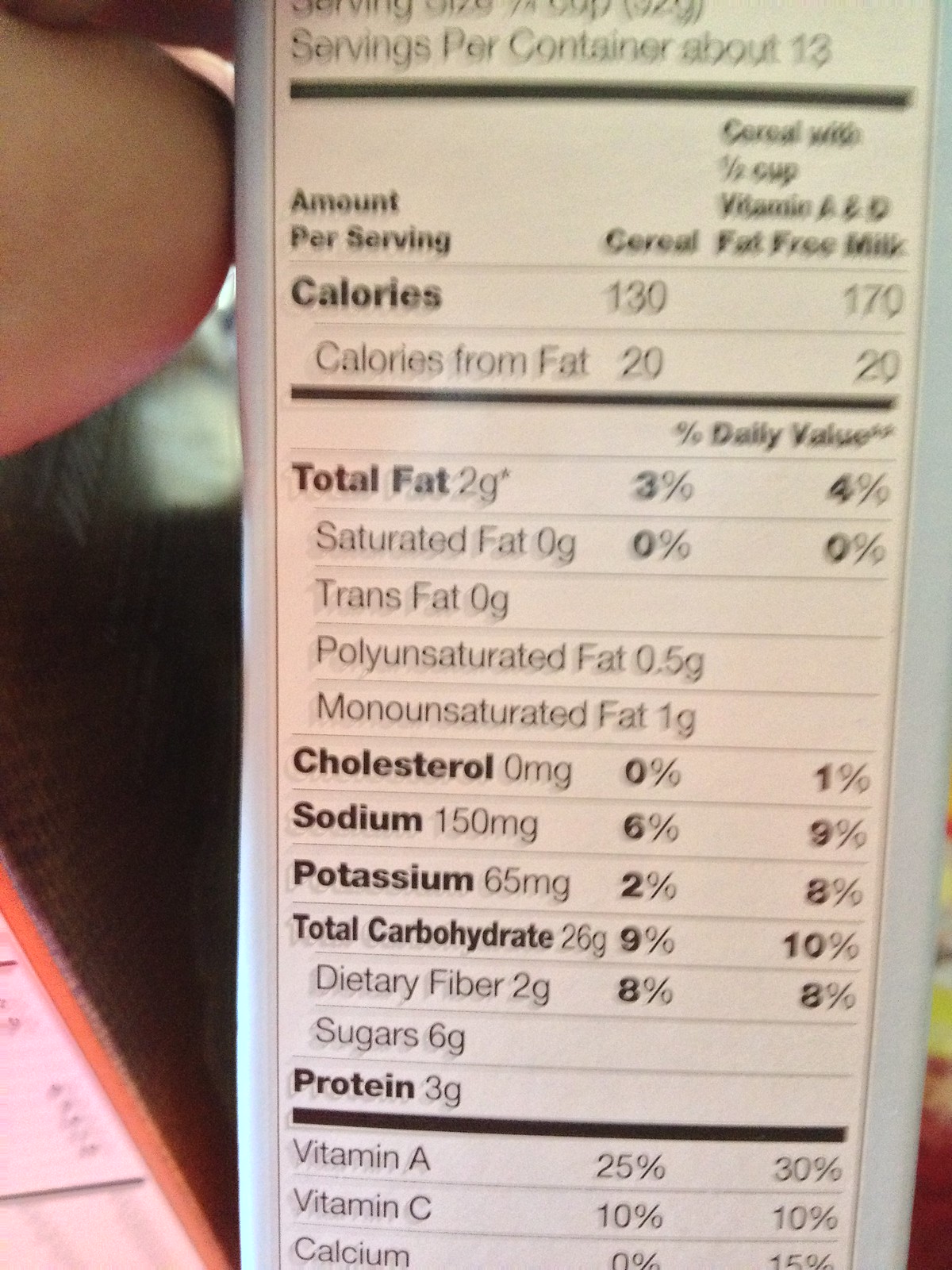The image is a close-up photograph of a nutrition label on a box, possibly cereal, with a fingertip holding the side of the box. The label is bordered in light blue and written in black on a white background. Although the image is slightly blurry and part of the label is cut off, most details are discernible. The label lists the nutritional content for both the cereal alone and with half a cup of vitamin A and D fat-free milk. It states there are about 13 servings per container. Each serving provides 130 calories (or 170 with milk), with 20 calories from fat. The total fat content is 2 grams (3% of the daily value) or 4% with milk, consisting of zero grams of saturated and trans fats, 0.2-0.5 grams of polyunsaturated fat, and 1 gram of monounsaturated fat. There is no cholesterol, translating to 0% of the daily value (but 1% with milk). Sodium is 150 milligrams (6% or 9% with milk), potassium 65 milligrams (2% or 8% with milk), total carbohydrates 26 grams (9% or 10% with milk), dietary fiber 2 grams (8%), sugars 6 grams, and protein 3 grams. Additionally, the vitamins and minerals listed include 25%-30% of vitamin A, 10% of vitamin C, and 0%-15% of calcium, depending on whether the cereal is consumed with milk.